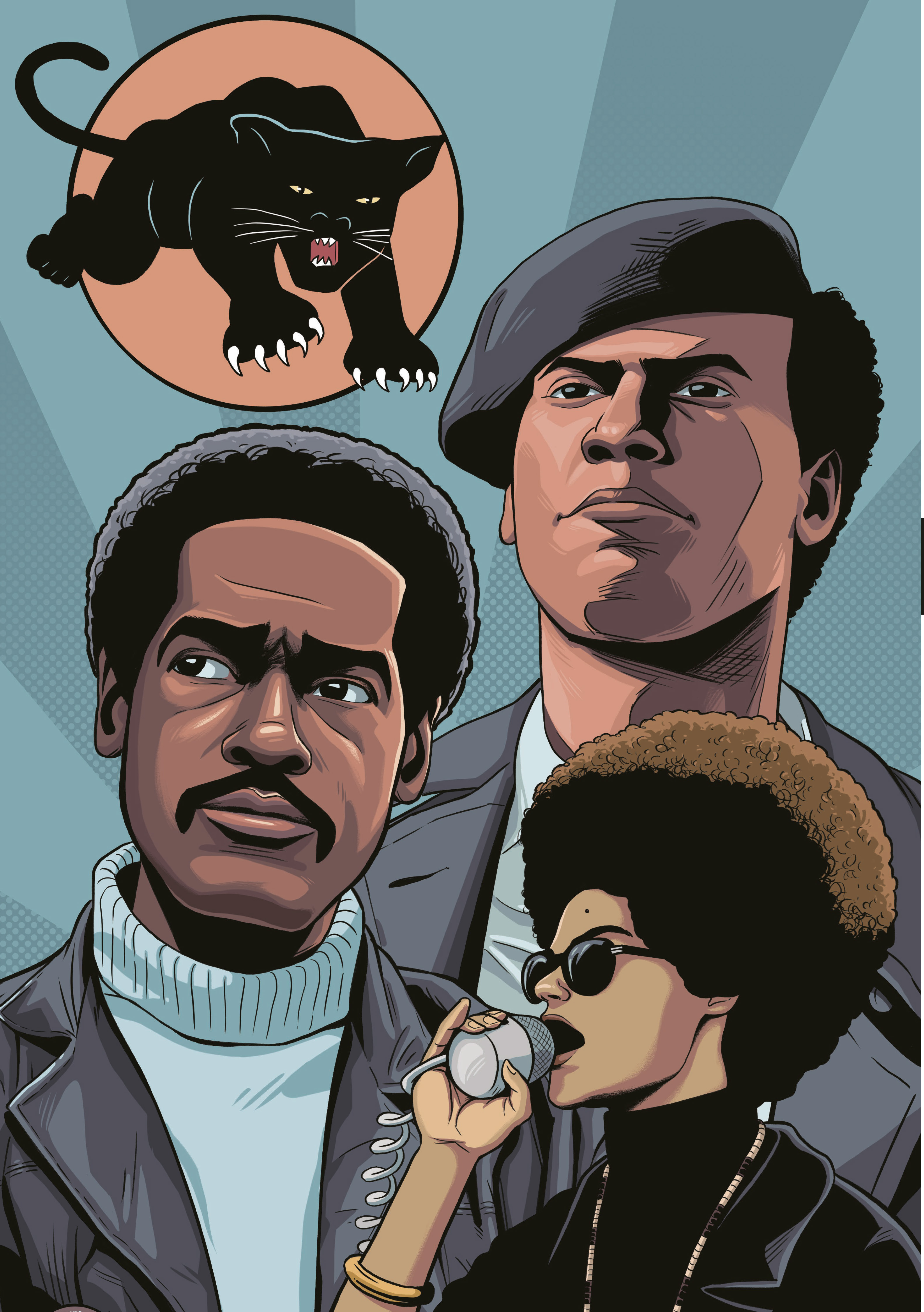This detailed pixel art combines elements of both a digital poster and comic book-style illustration, primarily featuring a group of Black Panthers. In the upper left corner, there is a black panther logo outlined in black against a salmon or peach-colored circle, depicting the panther with its claws out and mouth open. The background showcases a dynamic sunburst pattern with radiating shades of blue, teal, and gray.

Foregrounding the scene are three African Americans in iconic Black Panther attire. On the left stands a man with a short afro, mustache, wearing a light blue turtleneck under a brown or dark jacket. Next to him is another man, larger in size, wearing a black beret, and a light blue button-down shirt beneath a dark jacket, looking up seriously. In the front right corner is a striking representation of Angela Davis in profile, her large afro framing black sunglasses and a passionate yet serious expression as she speaks into a microphone. She is dressed entirely in black, completing the powerful composition of this vibrant, poignant artwork.